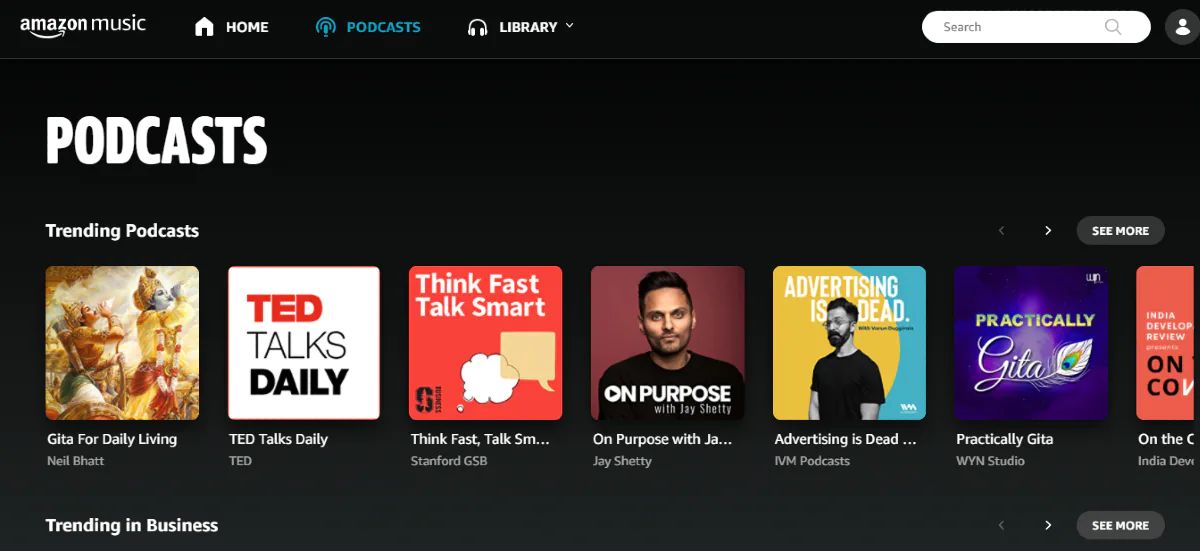This image is a screenshot from the Amazon Music website, set against a black background and oriented horizontally. In the upper left corner, the Amazon Music logo is displayed in white. Beneath this, a navigation bar includes a home icon labeled "Home," a blue section for "Podcasts," and a "Library" tab featuring a headset icon and a drop-down menu.

On the upper right side, there is a white search bar adjacent to a generic profile image. Dominating the central portion of the image, large white text reads "Podcasts," with "Trending Podcasts" listed immediately below. Several podcast covers are partially visible, including titles such as "Gita for Daily Living," "TED Talks Daily," "Think Fast, Talk Smart," and "On Purpose with Jay Shetty." Additional titles like "Advertising is Dead," "Practically Gita," and one starting with "Onco" in black letters on a red background, are also shown, though the latter is cut off due to screen space.

At the top and bottom of the podcast list, white "See More" text indicates that additional content can be viewed by scrolling or clicking the respective links. A partially visible section titled "Trending in Business" is also cut off at the bottom of the image.